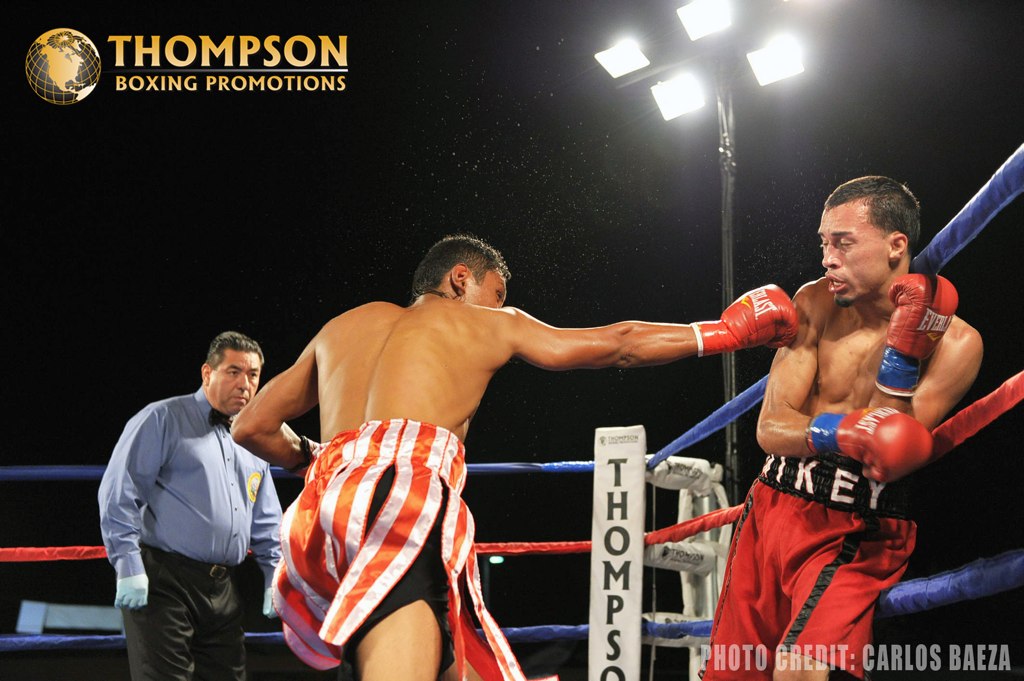The photograph captures an intense moment during a boxing match under the lights. In the center of the ring, two boxers are engaged in combat. The boxer on the left, mid-punch, is wearing white shorts with orange and black stripes and red boxing gloves. His opponent on the right, who is leaning against the ropes and bracing for the impact, dons orange shorts with a red stripe that say "Mikey" around the waistband. His gloves, also red, are emblazoned with "Everlast."

To the left of the action stands the referee, who is focused intently on the fight. He wears a blue button-down shirt, black dress slacks, a black bowtie, and rubber gloves. The referee appears slightly overweight and very serious.

Above the action, four lights illuminate the ring, highlighting the drama of the night match. In the top left corner of the image, the text reads "Thompson Boxing Promotions" alongside a small globe logo. The bottom right corner features a watermark crediting the photo to Carlos Baez.